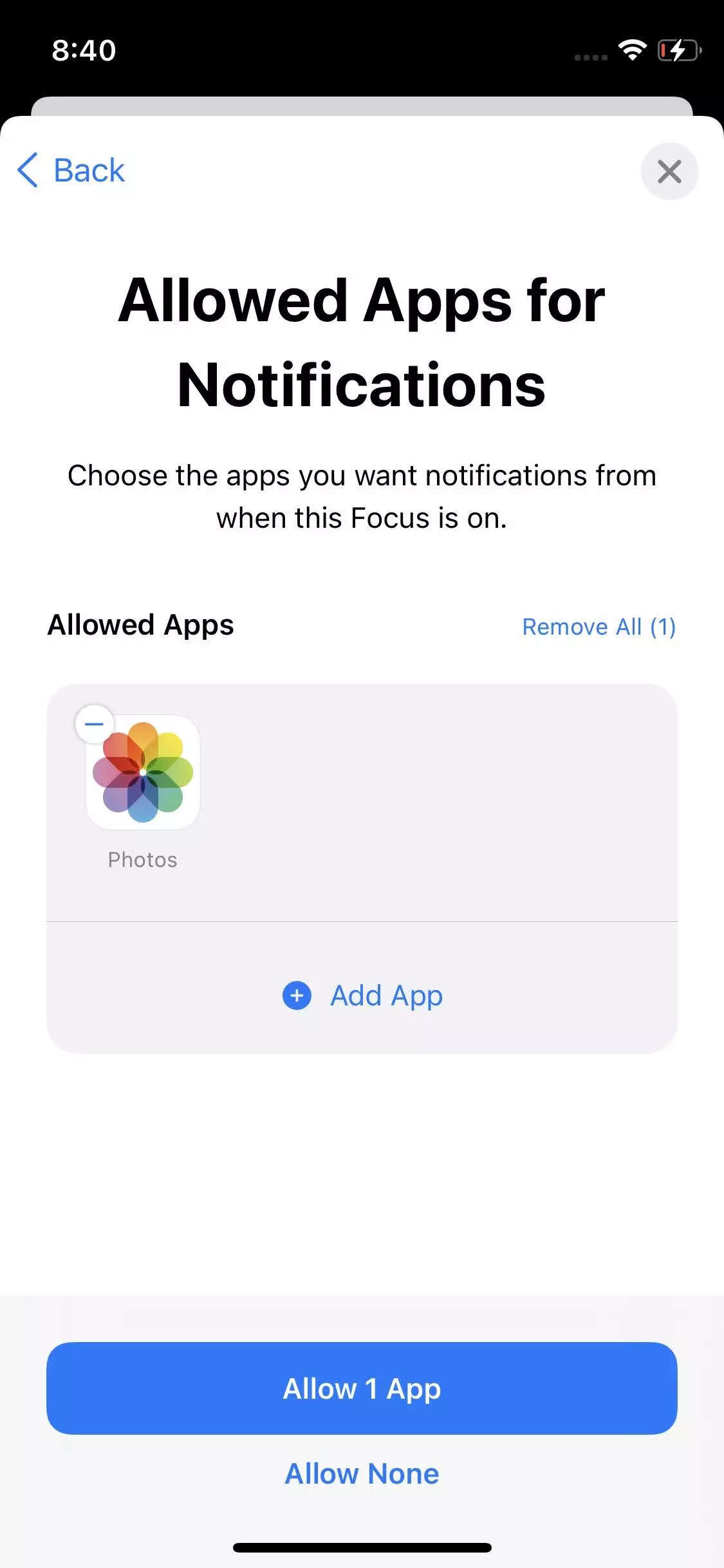The image features a detailed interface of a notification settings screen. At the top of the image, the background is black. In the upper left corner, there is a white text displaying "8:40," indicating the time. Adjacent to this on the right, a white Wi-Fi signal icon is visible, signifying a Wi-Fi connection. To the far right, there's a battery icon with a sliver of red, signaling that it is low but currently charging, as indicated by a white lightning bolt symbol over it.

The background transitions to white on the left-hand side where the tail end of a blue arrow is visible, pointing left, with the word "Back" in blue and a capital "B." On the opposite side, there is a gray circle containing a darker gray "X," likely serving as an exit or close button.

Centered in the middle of the image, bold black text reads "Allowed apps for notification." Below this heading, in a smaller black font, it says, "Choose the apps you want notifications from when this focus is on." Further down, another bold black heading states "Allowed apps," with a blue "Remove apps (1)" option next to it.

Underneath this section, there is a gray rectangle with the text "Photos" in gray. Above this text, there is a white square featuring a rainbow-colored flower icon. A thin gray line separates this area from a blue circle on the right, which contains a white plus sign, symbolizing the option to "Add." Next to it, blue text says "Add app."

Padding out the bottom portion of the image is a light gray rectangle. At the top of this rectangle, a long blue button displays the word "ALLOW" in white capital letters. Below this blue button, in blue text, it says "Allow apps." Further down in the same blue text, it states "Allow None," both phrases starting with capital letters. A black line runs horizontally, demarcating the bottom of the interface.